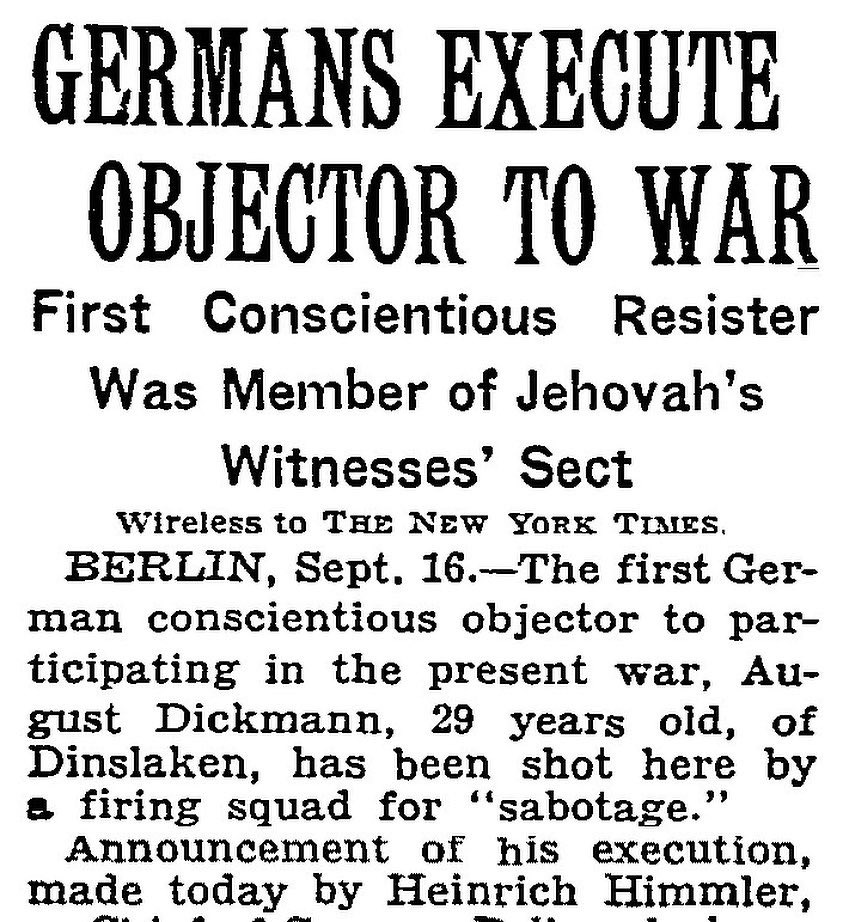The image depicts a scan or printout of an old-fashioned newspaper article likely from the 1940s, during World War II. The headline is prominently displayed in large black text, reading, "GERMANS EXECUTE OBJECTOR TO WAR." Directly below, a subheading states, "First conscientious resistor was a member of Jehovah's Witness sect." The article signifies its source with "Wireless to the New York Times." The main text begins: "Berlin, September 16th – The first German conscientious objector to participate in the present war, August Dickman, 29 years old, of Dinslaken, has been shot here by a firing squad for 'sabotage'." A new paragraph mentions the announcement of his execution, made by Heinrich Himmler, although the article is cut off at this point. The background is white, and the text is in a distinctive, old-fashioned font. The article does not specify the year, but given Heinrich Himmler's involvement, it is likely from World War II. No images are included, and the date is only mentioned as September 16th.